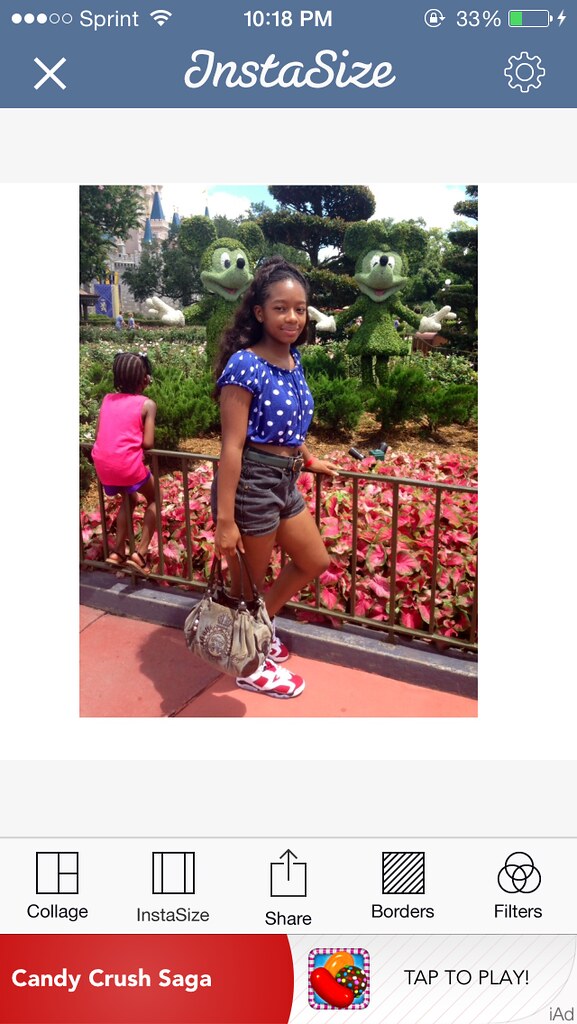The screenshot from a mobile phone shows a detailed and vivid scene. At the top of the screen, a blue banner with white text displays phone statistics, including "Sprint," a Wi-Fi icon, "10:18 PM," and "53%" inside a green battery outline. Directly below, we can see three icons: an "X," the app name "Instasize" in white cursive text, and a gear wheel. The main part of the image features two young girls posing at a theme park. The older girl, a young Black woman or teenager, is wearing a blue crop top with white polka dots, blue or gray denim shorts, and a belt. She holds a cream-colored bag in her right hand and a metal railing with her left, behind which are topiary figures resembling Mickey and Minnie Mouse, as well as the Magic Kingdom castle in the background. The younger girl, dressed in a pink sleeveless top and purple shorts, is leaning over the railing, looking back at the topiary figures. The setting includes colorful red leaves and plants around the railing. At the bottom, the app interface shows five buttons labeled "Collage," "Instasize," "Share," "Borders," and "Filters," along with an ad for "Candy Crush Saga" that invites users to tap and play.